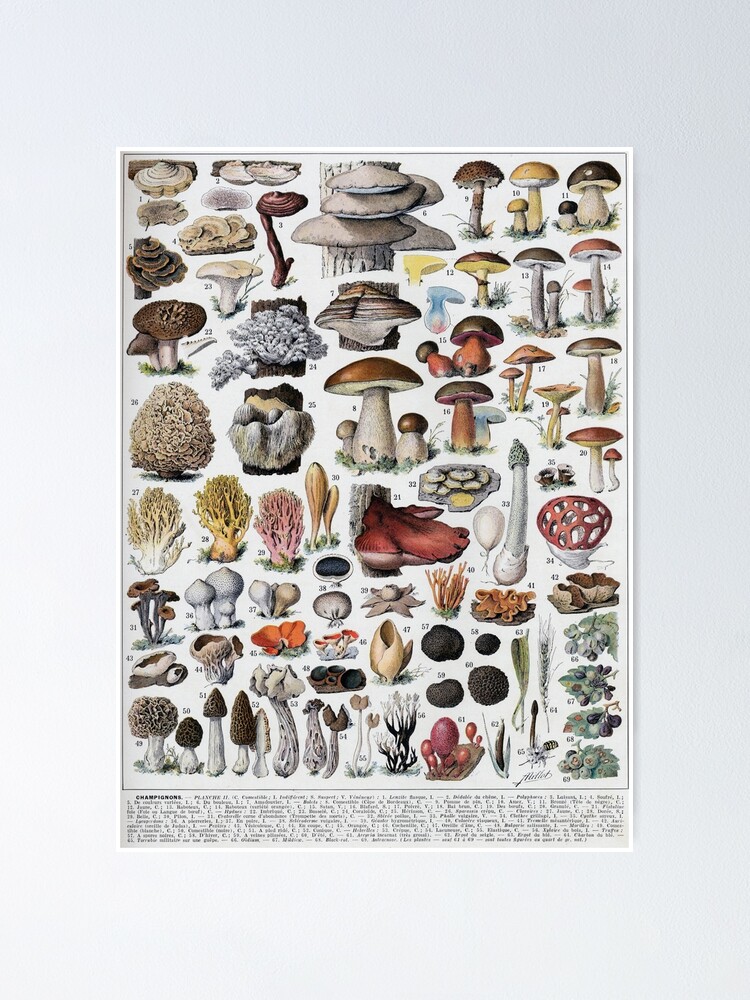This visually detailed science poster showcases approximately 100 different types and varieties of mushrooms, all meticulously illustrated in their natural state. The artwork employs a palette of realistic colors, including various shades of browns, tans, whites, reds, yellows, oranges, grays, greens, pinks, and even blues, representing the vibrant diversity found in nature. Each mushroom, whether tall, short, or uniquely shaped, is numbered, and these numbers correspond to detailed descriptions provided in small print at the bottom of the poster.

Some of the mushrooms are depicted growing out of wood and attached to trees, which are also drawn into the scene, emphasizing their natural habitats. The poster includes a wide array of mushrooms such as morels, toadstools in various sizes, conch, coral-type fungi, and many others, making it an exhaustive illustrated reference.

The background of the poster is white, providing a clean contrast to the colorful mushrooms, and it is bordered by a light blue mat around the image and bordered additionally with a gray mat, giving it a framed and polished look. This poster, reminiscent of a scientific chart you might find in a high school science lab, serves as an informative and aesthetically pleasing guide for identifying and learning about different mushroom species.